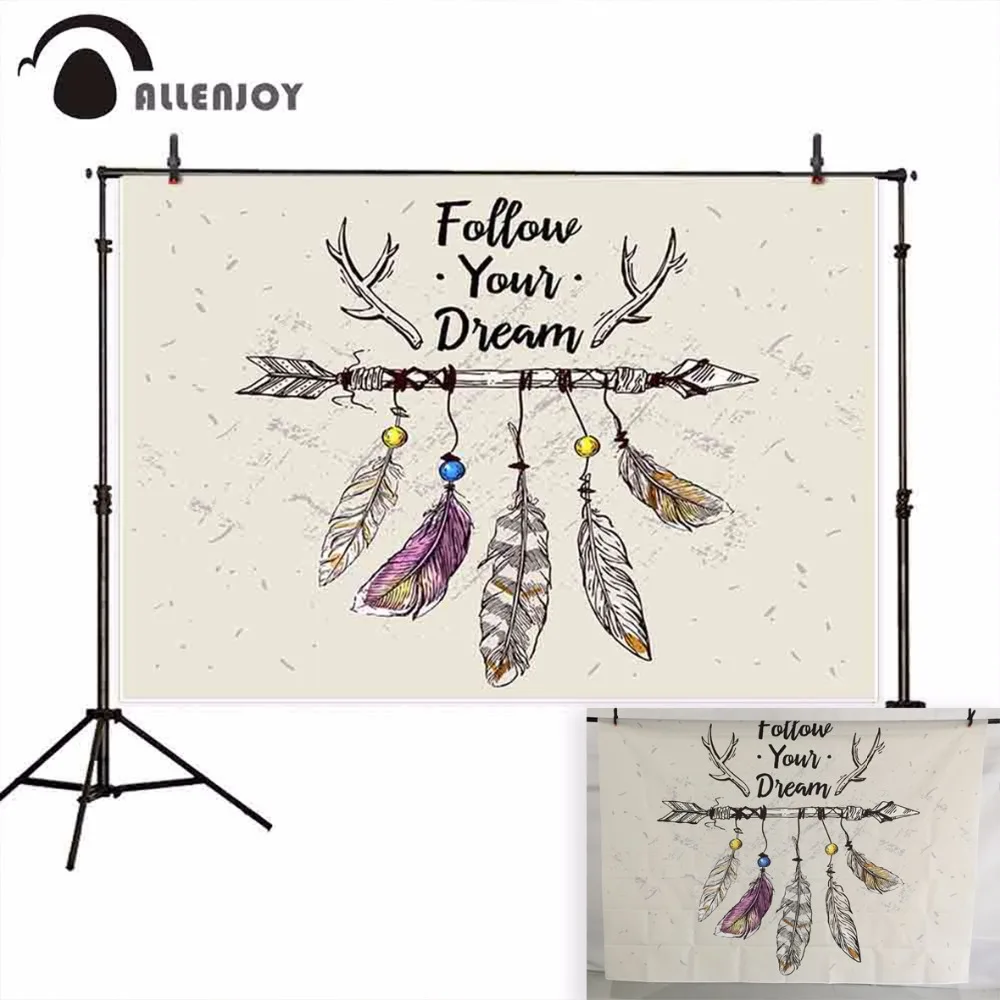This image appears to be an advertisement, likely from a catalog, showcasing a photography backdrop. The backdrop is mounted on a telescoping pole system with tripod legs on either side, and the entire setup is against a white background, emphasizing its standalone display. At the top center of the image, there is a logo that reads "Allenjoy," suggesting the brand or website.

The main visual element is a large, parchment-colored poster held by black clips attached to the pole system. The poster features the inspirational phrase "Follow Your Dream" written in elegant cursive at the top. Framing the text are detailed illustrations of deer antlers on either side. Below the text, a Native American-style arrow stretches horizontally, decorated with five feathers hanging from strings. Each feather is adorned with small beads—with two yellow beads, one blue bead, and the remaining feathers primarily showcasing neutral colors such as black, white, and brown. One feather is particularly vibrant with hues of purple and yellow.

Additionally, in the bottom right corner of the image, there is a smaller inset photo. This close-up shot replicates the main backdrop in a real-life setting, providing a tangible example of the product's application. The detailed and colorful artistic elements, combined with the functional tripod setup, make this backdrop both visually appealing and practical for photography purposes.